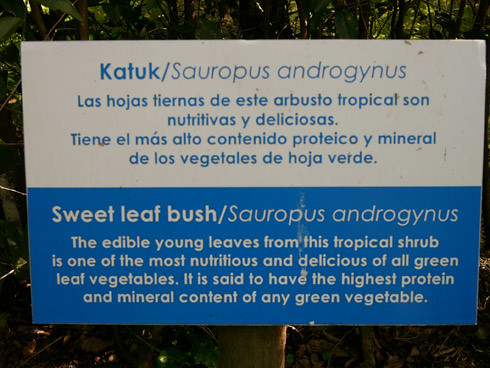The image depicts an outdoor rectangular sign mounted on a wooden post, surrounded by green foliage and vegetation. The sign is divided horizontally, with the top half featuring white background and blue text, and the bottom half showcasing a blue background with white text. The upper section is written in a language that appears to be Spanish, while the bottom section is in English. The English portion reads: "Sweet Leaf Bush (Sauropus androgynus): The edible young leaves from this tropical shrub are among the most nutritious and delicious of all green leafy vegetables. It is said to have the highest protein and mineral content of any green vegetable." The informational sign emphasizes the nutritional qualities of the sweet leaf bush and is rendered in a bold, sans serif font, reminiscent of Century Gothic.